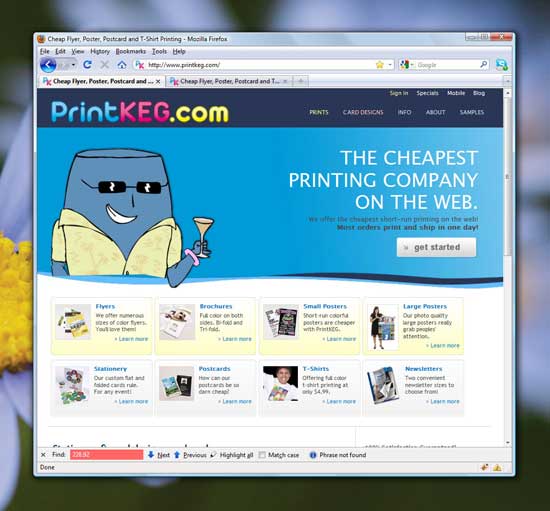The image displays the "PrintKega.com" website, as seen in the Firefox web browser. The familiar Firefox logo is visible in the upper left-hand corner of the window. At the top of the webpage, the site's name is prominently shown with "print" in blue text, "KEG" in bold red capital letters, and ".com" in yellow.

A navigation menu is situated underneath the site name, featuring tabs labeled "Prints," "Card Designs," "Info About," and "Samples." Above this menu, there is a small sign-in button for returning users.

The main banner of the site showcases a stylized human figure with blue skin, wearing sunglasses, a flat-topped head, and a yellow shirt. The figure has a playful smirk and is holding a martini glass in its left hand. To the right of this figure, the slogan "The cheapest printed company on the web" is clearly displayed, emphasizing the company's commitment to affordable printing services.